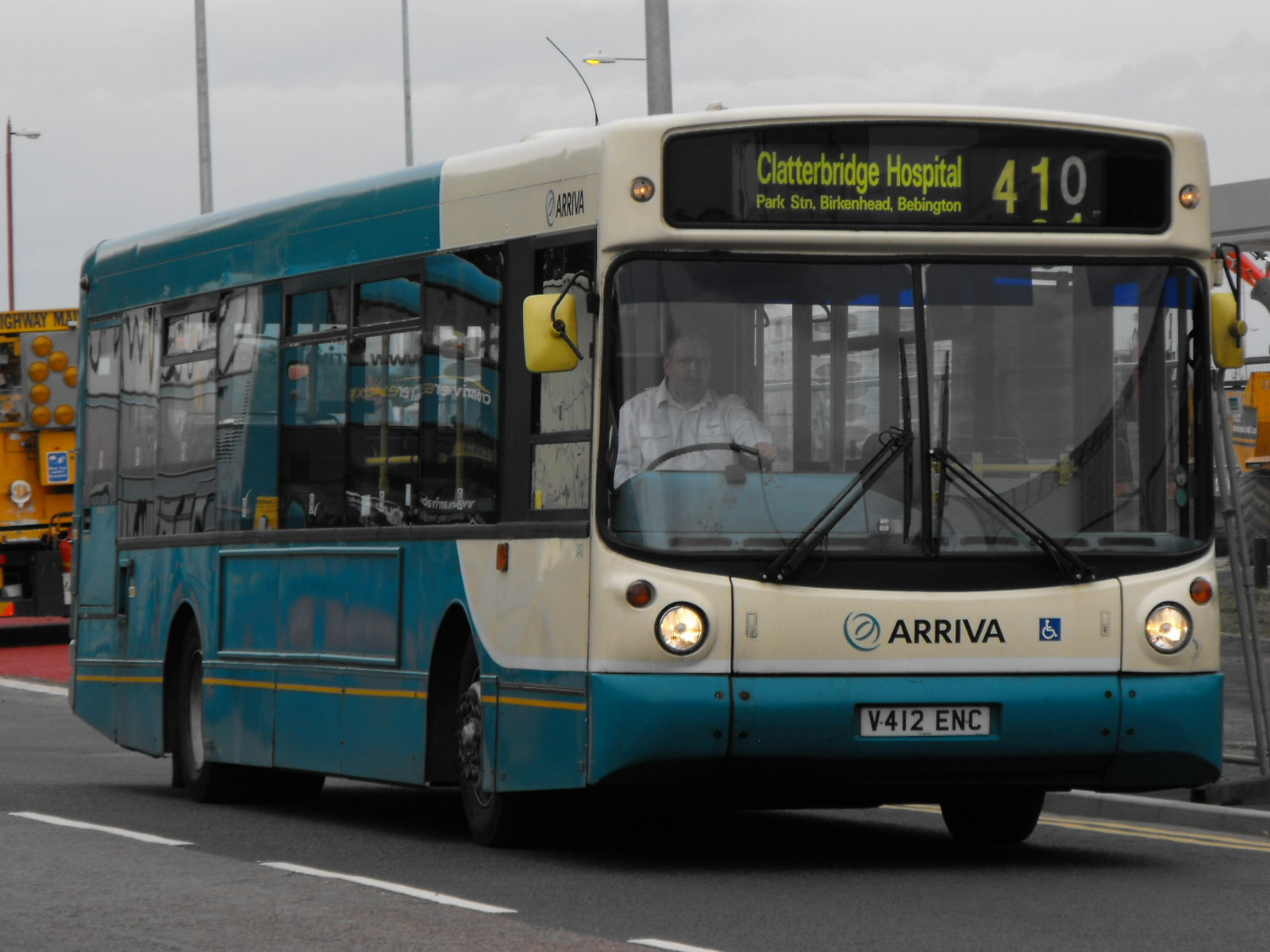The image depicts an older model city transit bus, adorned primarily in a darker teal blue with white embellishments on the front and part of the left side. The bus, notable for its flat front end, is captured outdoors on an overcast day, suggesting it is likely in the UK, given the right-hand side driver's position. The driver, a Caucasian man wearing a white button-up shirt, is visible through the front glass. Above the windshield, a black sign in greenish-yellow print lists the bus's route: Clatterbridge Hospital, Park Station, Birkenhead, Bevington, designated as number 410. The bus appears to be in good shape despite its age and currently has its headlights on. The lettering "Arriva" is printed in black at the center bottom of the front face. An orangish bus is visible behind it, adding context to the urban setting.